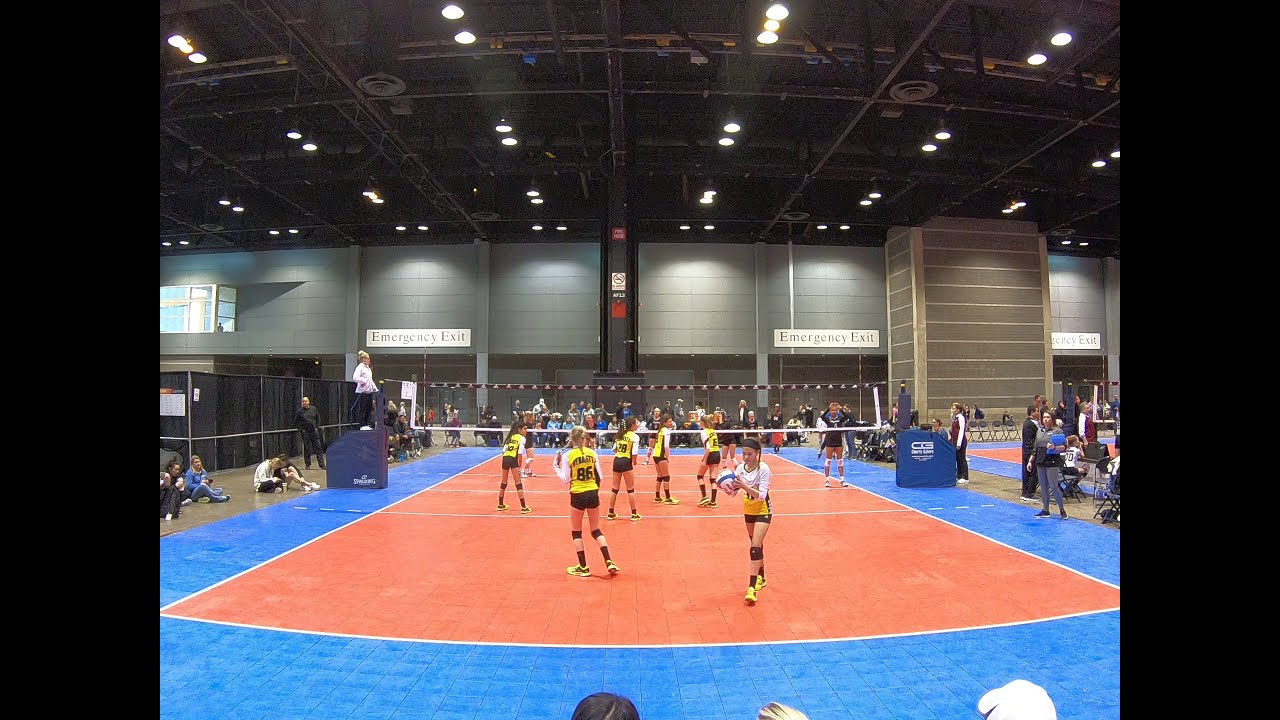The photograph captures an action-packed moment in an indoor women's volleyball tournament held in a large, open gymnasium with tall ceilings and an unfinished metal framework visible overhead. The main focus is on one side of the court, where a player from the team in yellow jerseys with black shorts is walking back to the baseline, preparing to serve. The court itself has a rust-colored playing area bordered by bright blue. 

Spectators fill the stands in the foreground, with the tops of a few heads visible, and more spectators can be seen seated across the net and to the left and right sides of the court. There is a referee positioned on a podium to the left side of the net, while another official stands behind another podium on the right. The background wall features emergency exit doors clearly labeled in multiple languages. Also, on the back wall is a scoreboard on the upper left and other signs that appear to indicate additional exits.

Signs of a second volleyball court are visible in the upper left corner of the photograph, hinting at the facility's capacity to host multiple games simultaneously. The bright lighting from the ceiling illuminates the ongoing game, adding to the energetic atmosphere of the competition.